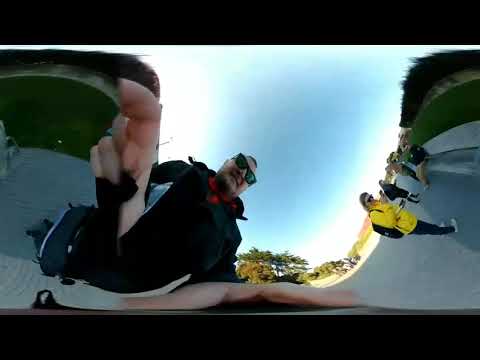The image captures a middle-aged man, likely in his 40s or early 50s, taking a selfie from a low angle, looking up into his face. He has a balding head and wears sunglasses alongside a worn-rimmed pair of spectacles. He's dressed in a black jacket, possibly zipped up, with a black checkered scarf and a red hoodie draped around his shoulders. The scene behind him features several people skewed to the right side due to heavy distortion—some standing, others seated on a cement bench that borders the asphalt road. One noticeable woman nearby sports a green parka and carries a backpack. The background is comprised of a sidewalk accompanied by greenery, including bushes and trees, under a blue sky adorned with thin white clouds. The image's perspective and distortion make the surrounding elements, like the trees to the left and the road bordered by hedges, appear tilted.